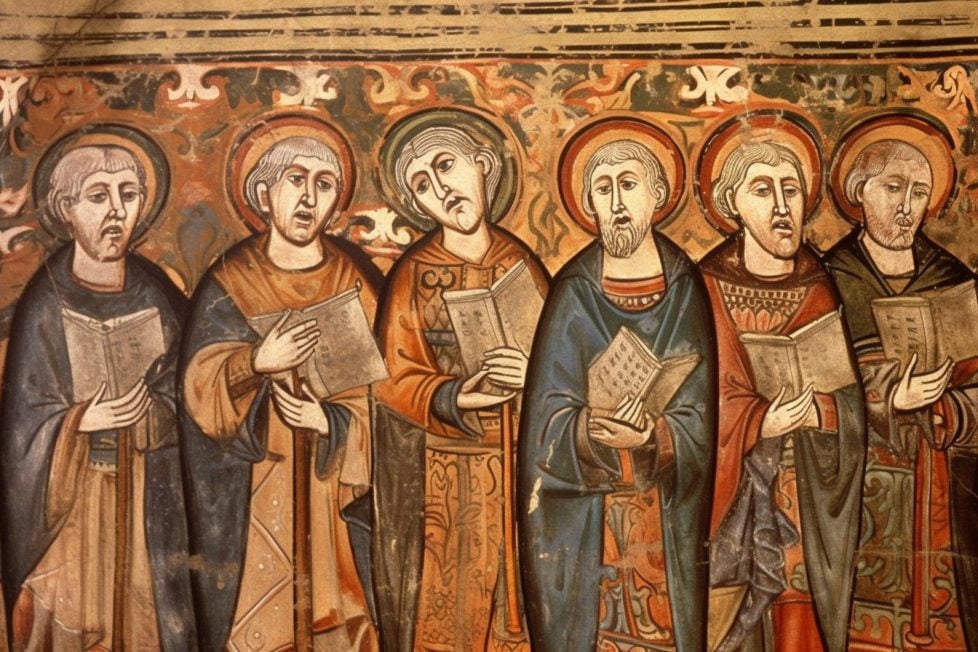The image is a richly detailed painting reminiscent of Medieval or Renaissance art, portraying six elderly holy men, possibly monks, friars, or priests, vested in robes and engaged in what appears to be singing or conversing. The men each have white hair and halos encircling their heads, indicating their sanctity. They are arranged in a row, each holding an open holy book or hymnal. From left to right, their robes vary in color: the first, second, and fourth men are dressed in blue; the third in gold; the fifth in red; and the sixth in green. The background features a decorative pattern resembling frescoed wallpaper, typical of the era's artistic style, predominantly depicted in muted, earthy tones with some splashes of blue. The men display a variety of expressions, with two of them sporting beards, specifically the one in the middle right and the one on the far right. Their arrangement and demeanor suggest a ceremonial or devotional setting pertaining to Christian or Catholic traditions.